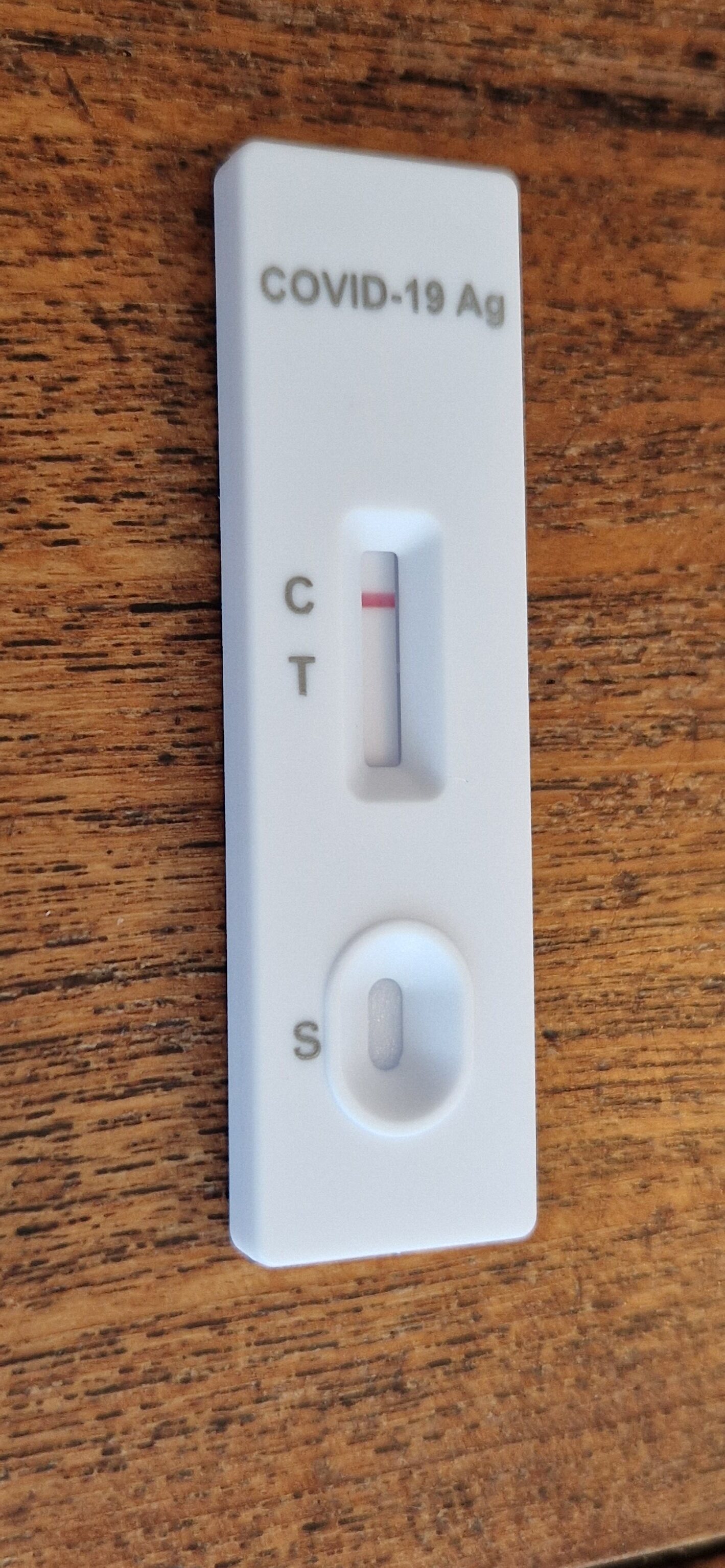In the image, a COVID-19 rapid antigen test is prominently displayed on a light brown, wood-grain tabletop flecked with black. The test is rectangular in shape and positioned vertically. Across the top, the text "COVID-19 AG" is clearly visible. Positioned centrally on the test, the letters "C" and "T" are marked to the left of a sunken rectangular window, within which a single red line appears next to the "C". At the bottom of the test, there is a circular indentation labeled with a capital "S". The image lacks any additional paraphernalia or explanations to interpret the test results. Taken from a left-hand side vantage point, the image is slightly blurry and features no other objects, capturing only the test against the wood-grain background.